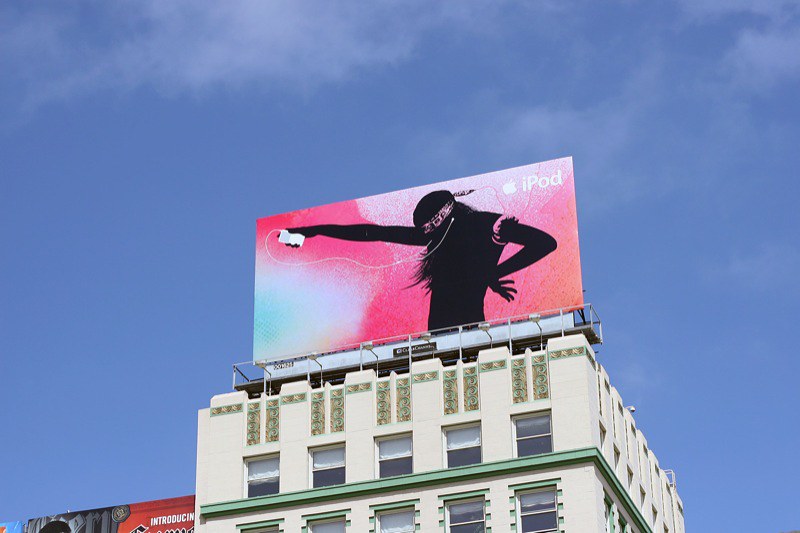The photograph, captured outdoors with a 45-degree upward angle, showcases a high-rise building crowned with a vibrant billboard. The building, emerging from the center bottom of the image, is white with a notable horizontal crane design and is adorned with a mix of rectangular and square windows. Green trim accents the structure, drawing the eye upwards to the billboard perched atop the building.

Dominating the upper right corner of the composition, the billboard prominently features the iconic bitten Apple logo in white, adjacent to the text "iPod". The advertisement displays a striking black silhouette of a person who is slightly bowed and wearing a backwards black baseball cap and a long-sleeve black shirt. The figure's right arm extends forward, holding a white iPod with the headphone cable elegantly curving back towards a white earbud nestled in their ear. A pink band wraps around the figure's left bicep, adding a splash of color that contrasts with the otherwise monochromatic silhouette.

The background of the billboard is a gradient of vivid pink and blue, blending harmoniously with the clear blue sky dotted with faint, wispy clouds. The stark contrast between the billboard's dynamic colors and the serene sky creates a visually arresting image, drawing attention to the sleek, modern design of the iPod advertisement. Another smaller, red and black billboard is partially visible in the bottom left of the image, hinting at the urban environment surrounding the high-rise.